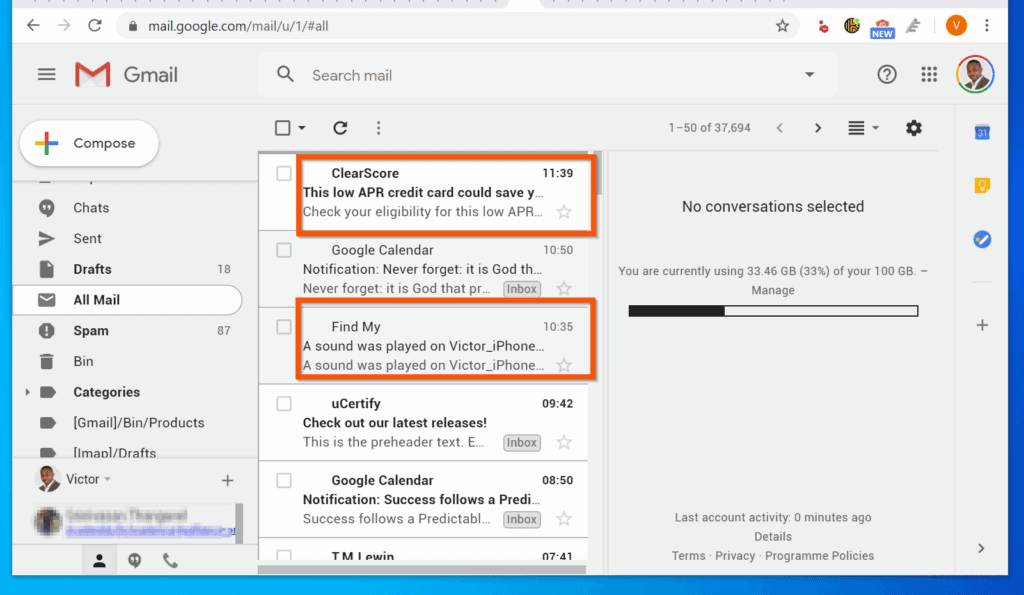**Detailed Caption:**

A screenshot of an individual's Gmail interface viewed in a web browser, specifically at the URL mail.google.com. At the very top of the screenshot, the URL is clearly visible, accompanied by several icons on the right side of the address bar. The interface has a predominantly gray theme typical of Gmail’s basic design.

The screen is divided into three columns. On the far left column, there is a "Compose" button, prominently displayed as a white button, allowing the user to draft new emails. Below this button, a list of folder options is visible, including "Inbox," "Sent," "Drafts," "All Mail," "Spam," and more. The "All Mail" option is currently highlighted, indicating it is selected.

The middle column displays a list of emails. Two emails are in focus, marked by red text; one is from "Clear Score" and the other from "Find My." These emails are circled, suggesting they may be flagged or otherwise highlighted.

The rightmost column serves as the email preview pane, currently stating "No conversation selected," indicating that no email is currently open for reading or preview.

At the top of the interface, just below the URL and icons, the Gmail logo and a search box are situated on the left, while on the right side of this bar, there is a color profile photo placeholder, showing the user's account profile.

The overall layout provides a user-friendly and organized view of the Gmail interface, with ample space for navigating folders, viewing email lists, and previewing email content.